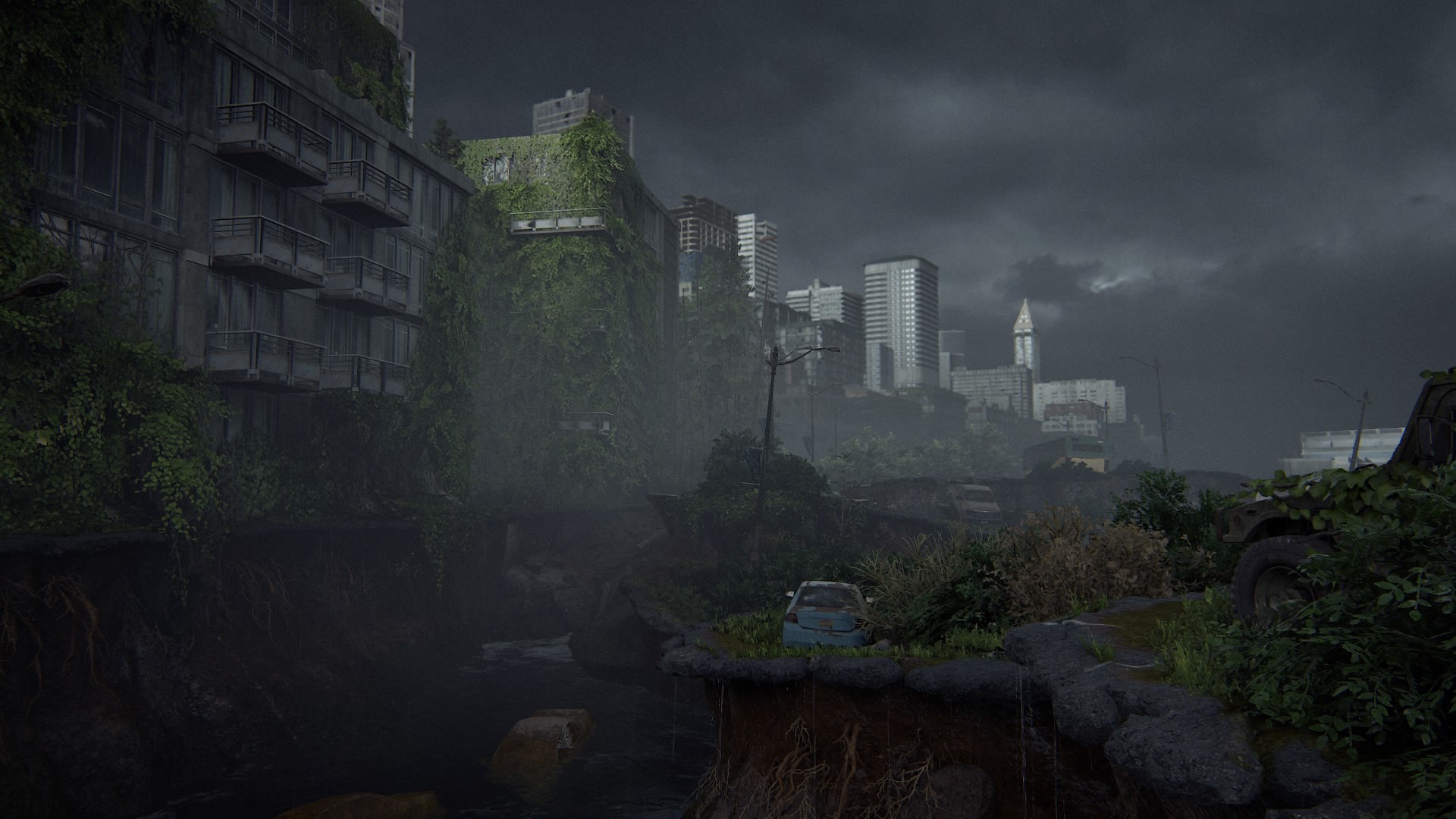This artwork, likely a painting, portrays a dystopian scene predominantly rendered in black and white, with selective elements of color. The focal point is a seemingly abandoned white sedan car parked precariously at the edge of a jagged, rocky cliff. Below, a desolate, dry riverbed is strewn with rocks and mud, accentuating the scene's bleakness. 

In the middle ground, a row of forsaken buildings stretches across the landscape, each structure bearing signs of abandonment and decay. An apartment building dominates the foreground, its empty balconies hinting at a once-thriving but now vacated existence. The building's charred facade suggests it may have endured a fire, adding to the somber, gray tone of the scene. Adjacent is a tall, derelict building almost entirely cloaked in moss and foliage, nature reclaiming the urban wasteland.

Further into the background, high-rise buildings stand solemnly under a sky heavy with menacing black clouds, despite the sun's fleeting rays casting a stark contrast. The tiny patches of greenery from grass and trees offer the only touch of color in this otherwise monochromatic and somber depiction of urban decay and abandonment.